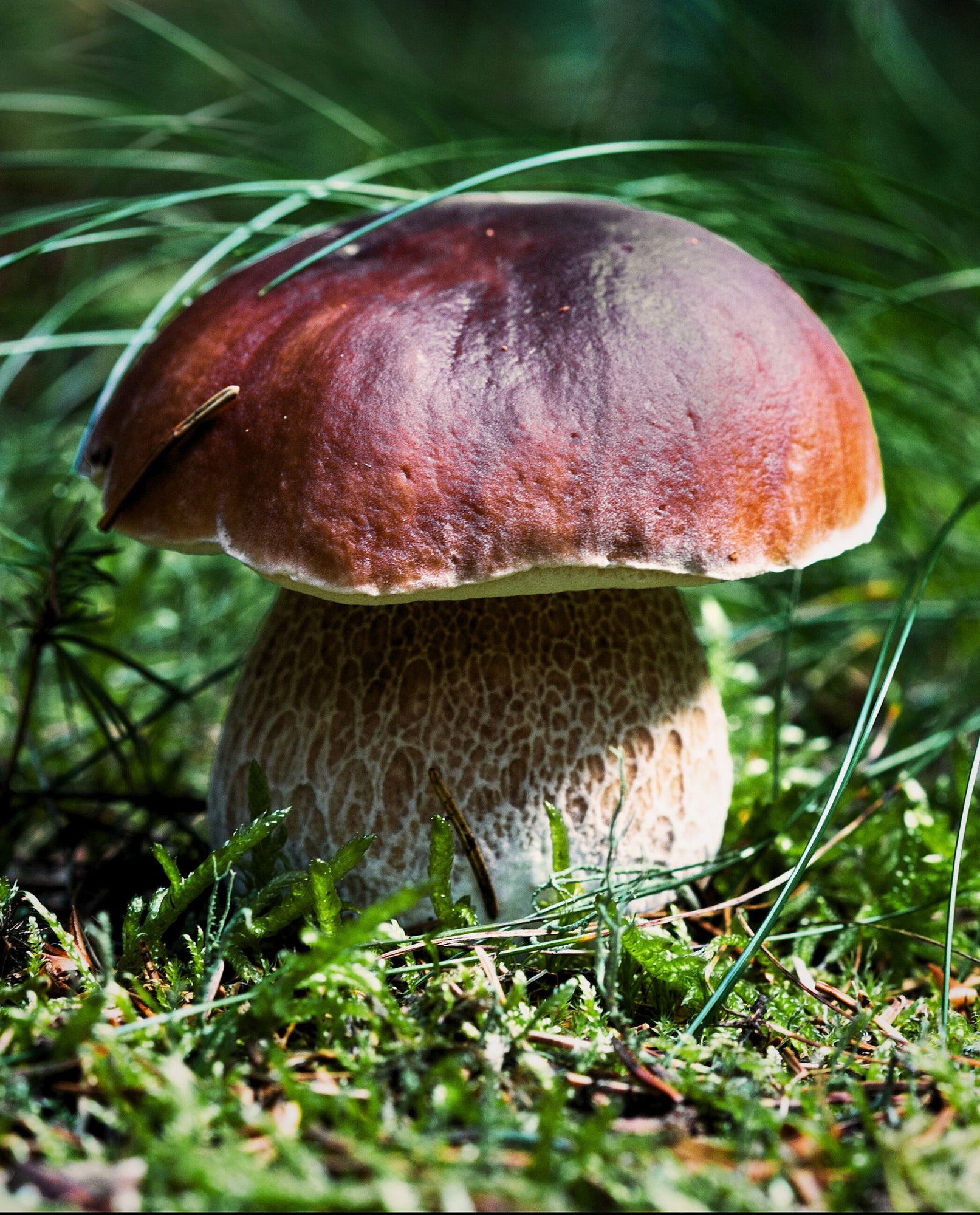This is a photograph of a very large mushroom growing outdoors amongst a lush, green landscape. The scene is dominated by long, thin blades of grass and green weed-like plants that surround and slightly arch over the mushroom. The mushroom's thick, oblong-shaped base is beige with a spongy, almost honeycomb-like texture and is streaked with white. Atop the base sits a substantial, round cap that displays a rich, orangish-maroon hue with some areas appearing darker. The mushroom looks robust, almost juicy, contrasting beautifully with the green, grassy surroundings. Nearby, small brown twigs and patches of brown speckled among the greenery add subtle earthy tones to the vibrant outdoor setting, evoking an image reminiscent of a scene from the Mario Brothers game.